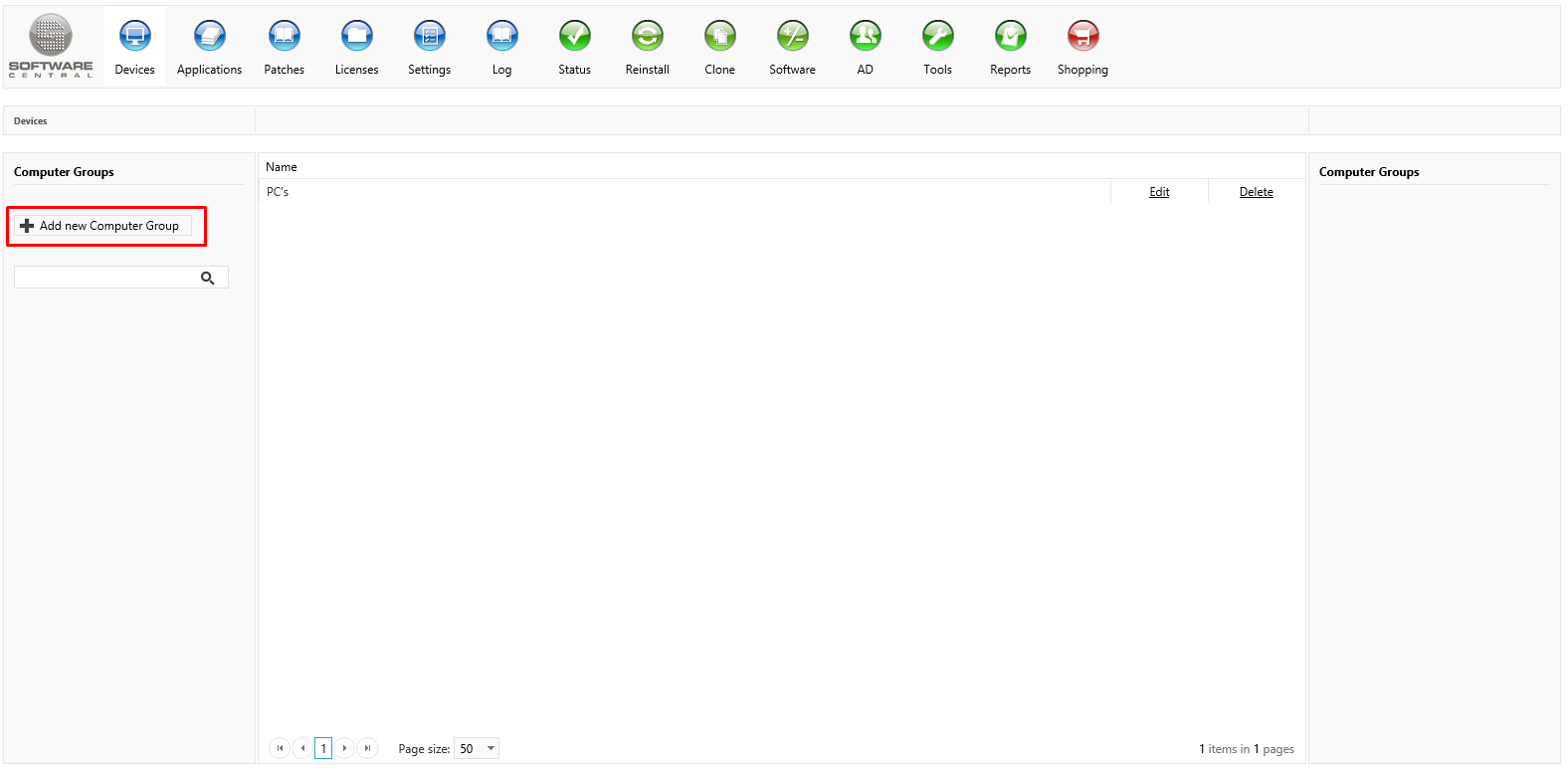The image displays a user interface with various elements partitioned across different sections. 

In the top left corner, there is an area representing software management which includes icons for devices, applications, and settings. Blue circles denoting growth, patches, licenses, and settings lock are prominently displayed. Adjacent to it, green circles indicate statuses such as reinstalling software, invoking support, identifying tools, reporting, and shopping. Additionally, there is signage for managing devices and computer groups.

A red-bordered section instructs users to "Add New Computer Group" and provides options to name, edit, or delete computer groups, typically labeled as "PCs." 

A textual note mentions "One item, so one page." 

On the bottom left, navigation controls include left and right arrows for pagination, distinctly marked with a blue border and the number 1, suggesting the current page. There is also a dropdown menu to select the page size, set to 15 items per page.

The center of the image features a white background, while the left side has a gray sidebar. This sidebar contains six blue circles, seven green circles, and one red circle, each likely representing different statuses or categories within the user's interface.

This detailed description reflects the organized and interactive elements of the software interface portrayed in the image.